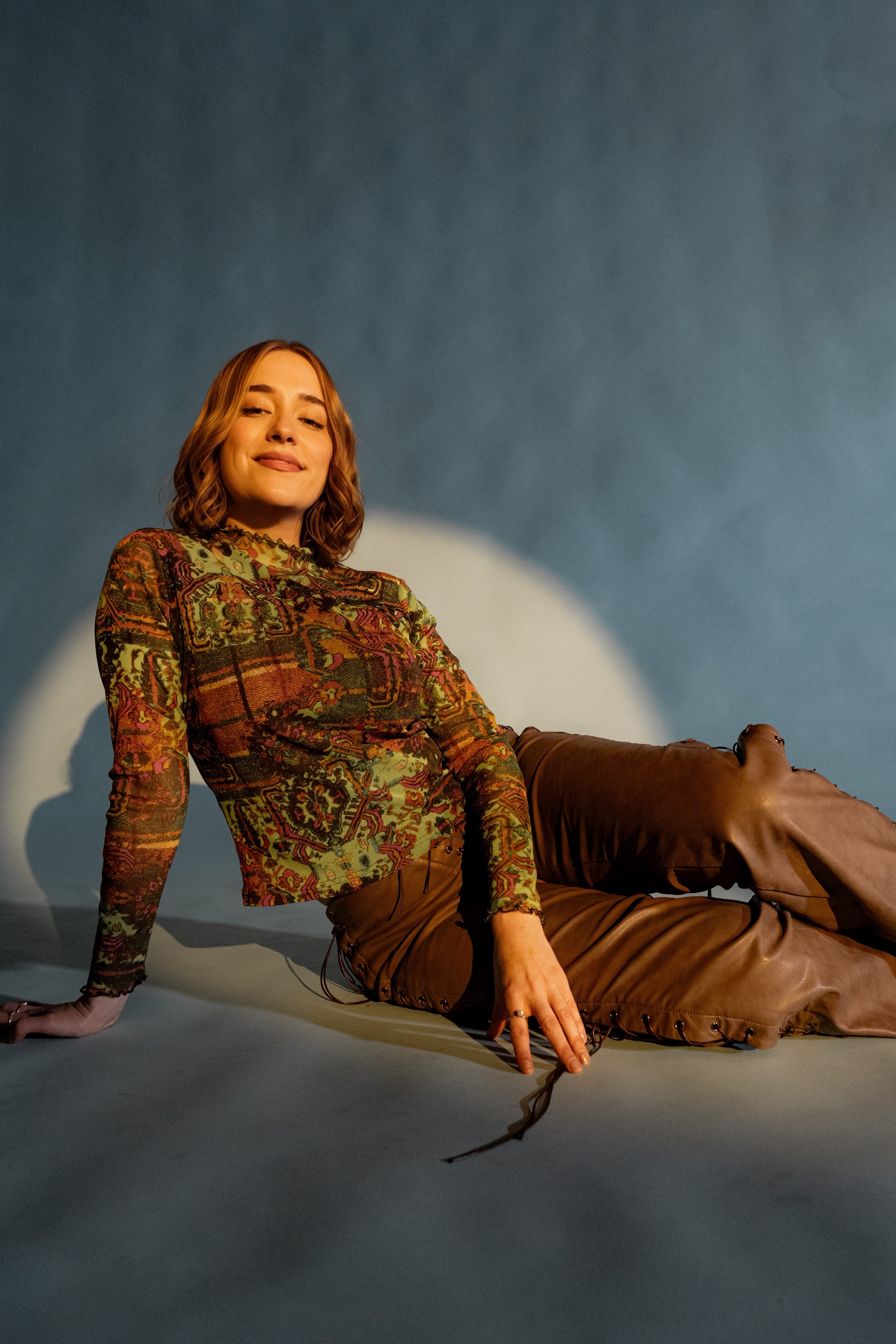In this studio photograph, a young European woman in her late twenties to early thirties is posed against a medium-blue grayish backdrop with a semicircle spotlight highlighting her upper body. She has shoulder-length reddish blonde hair parted in the middle and is smiling with her eyes half-closed, giving her a satisfied expression. Seated and slightly reclined on a grayish floor, she supports herself with her right arm while her legs stretch out to the side. She is dressed in muted fall tones that include a patterned blouse featuring greens, browns, and hints of orange and gold, paired with unique brown leather pants that tie up along the outer thighs. A silver ring adorns the index finger of her left hand.